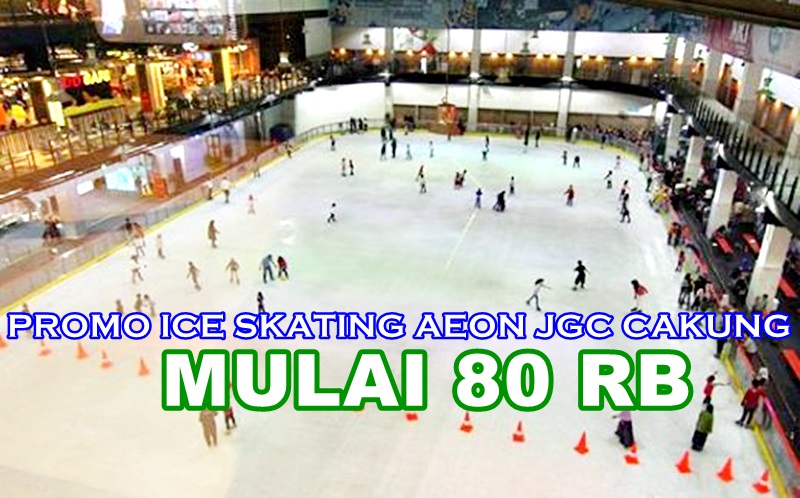The image is an aerial or elevated wide shot of an interior ice skating rink, capturing a dynamic scene with dozens of people skating on the ice. The rink is encircled by a walkway and has an additional level above it, featuring a series of lit rooms or sections divided by pillars. The rink resembles a pavilion, adding to its grandeur. Superimposed on the bottom half of the image is text written in white with blue and green highlights, reading "Promo Ice Skating AEON JGCKAKUNG." Below that, in larger letters, it states "MULAI 80RB."